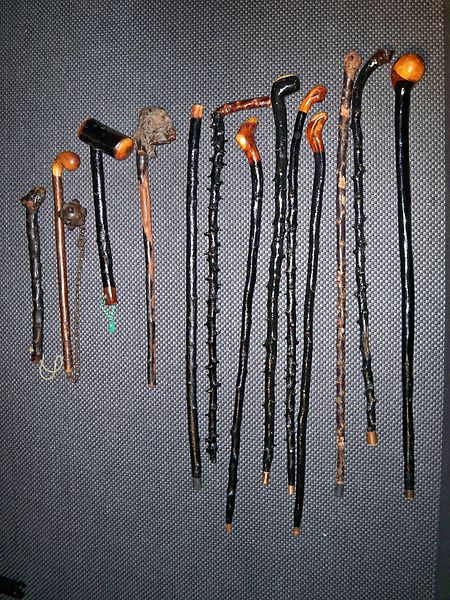Against a black, slightly textured background, a collection of walking sticks is arranged vertically from left to right. The background appears dark, with a subtle gradient where it's lighter in the center, creating a spotlight effect on the canes and walking sticks. The sticks display an intriguing variety in size and design, generally ordered from shortest on the left to longest on the right. Predominantly black in color, most have intricate wooden handles that introduce strokes of brown and orange into the scene. These handles vary greatly – some are circular, some knob-shaped, and one even resembles a monkey head. The sticks are not entirely straight, showcasing bumps and notches, and some incorporate unique features like a ball and chain or metal caps, adding to their distinctiveness and making a few appear as potential weapons. No people or text are present in the image, making the focus solely on the craftsmanship and diversity of the walking sticks.